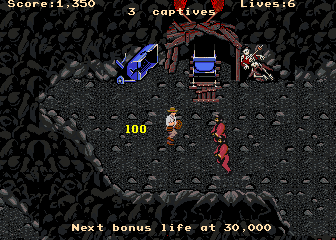This screenshot from a computer or video game captures a dynamic scene filled with intriguing details. At the top of the screen, there's a status bar displaying important information: "Score: 1350," "3 Captives," and "Lives: 6." Additionally, a message at the bottom informs the player, "Next bonus life at 30,000." 

The setting is a dark and ominous landscape, with the ground a mix of grey, dark grey, and black hues, adding to the eerie atmosphere. Three characters are central to the scene: a man sporting a brown top hat is engaged in conversation with two other characters dressed in red and black suits. In the background, the details deepen the mystery – a skeleton looms menacingly, the entrance of a cave beckons with potential secrets, and a blue wheelbarrow lies tipped over, suggesting recent activity or a past encounter.